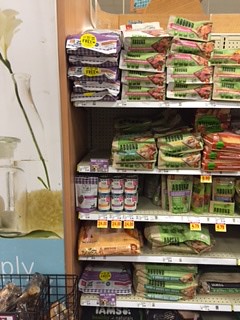This image showcases a grocery store aisle with a variety of products neatly arranged on shelves. On the left-hand side, there's a white wall, and in front of it, a plant with a long green stem and a white flower. At its base, there seems to be a sponge or similar object. Adjacent to the plant is a blue rectangular sign with white text, partially obscured by a shopping cart's edge. 

The right side of the image features grocery store shelving filled with numerous products. The top shelf contains purple packaged items on the left and green products on the right, with a red bag further down on the right. Beneath that, bags of different colors and sizes, including green and purple, are neatly stacked with some jars interspersed among the bags. The bottom shelf prominently displays a bag with the label "Iams," indicating dog food. Some of the bags appear to have Asian writing, suggesting they might contain rice or noodles, though it's difficult to ascertain due to the low image quality. Each shelf has price tags that are blurred and hard to read, further adding to the image’s low resolution.